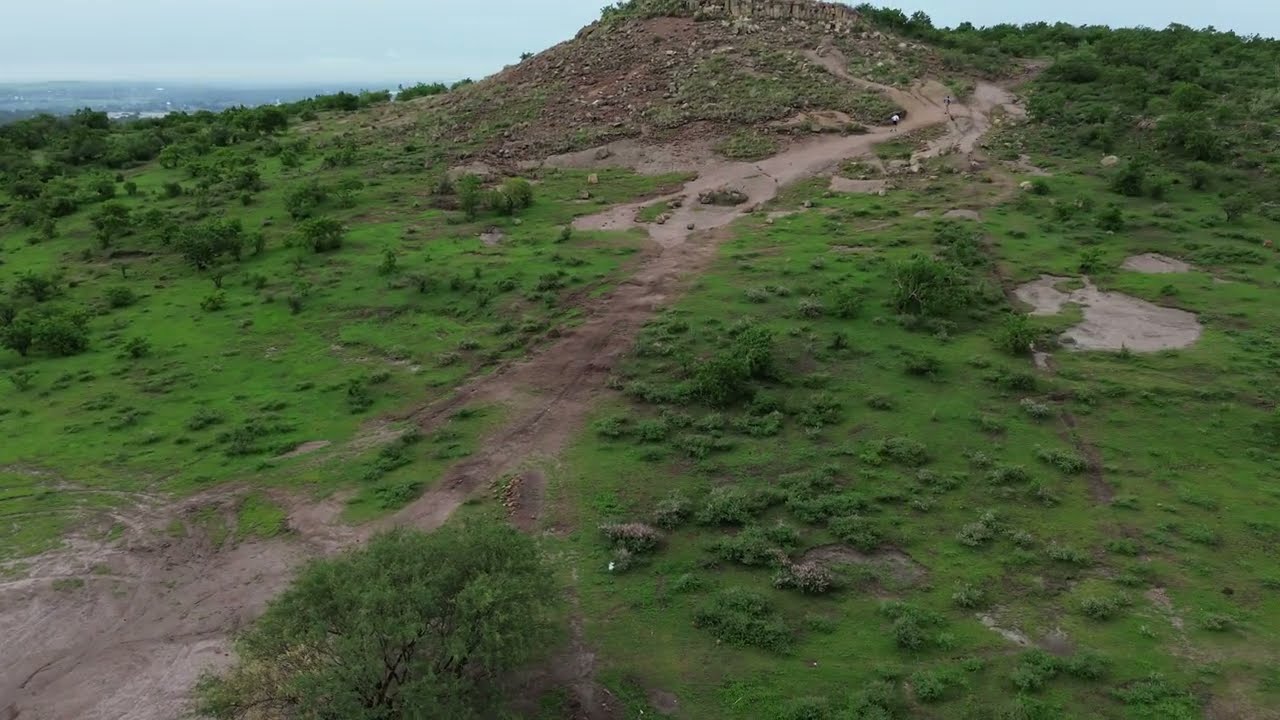This aerial daylight color photograph captures a well-traveled muddy dirt road that winds its way up a large, brown hillside, eventually reaching a rocky outcrop at the top. The road, grooved and marked with numerous tire tracks, starts from the bottom left corner, curving and ascending towards the top right area of the image. Alongside the path, patches of verdant green grass, low-lying bushes, and a few trees can be seen. A small, muddy circular pond is situated to the right of the trail. The surrounding landscape features a mix of green shrubs and scattered trees, contributing to a feeling of rustic terrain. In the distance, a misty horizon reveals a town with roads and buildings, under an overcast sky with shades of grayish blue and some smog. There is also a human figure wearing a white shirt and black pants standing on the path near a bend, adding a sense of scale to the scene.